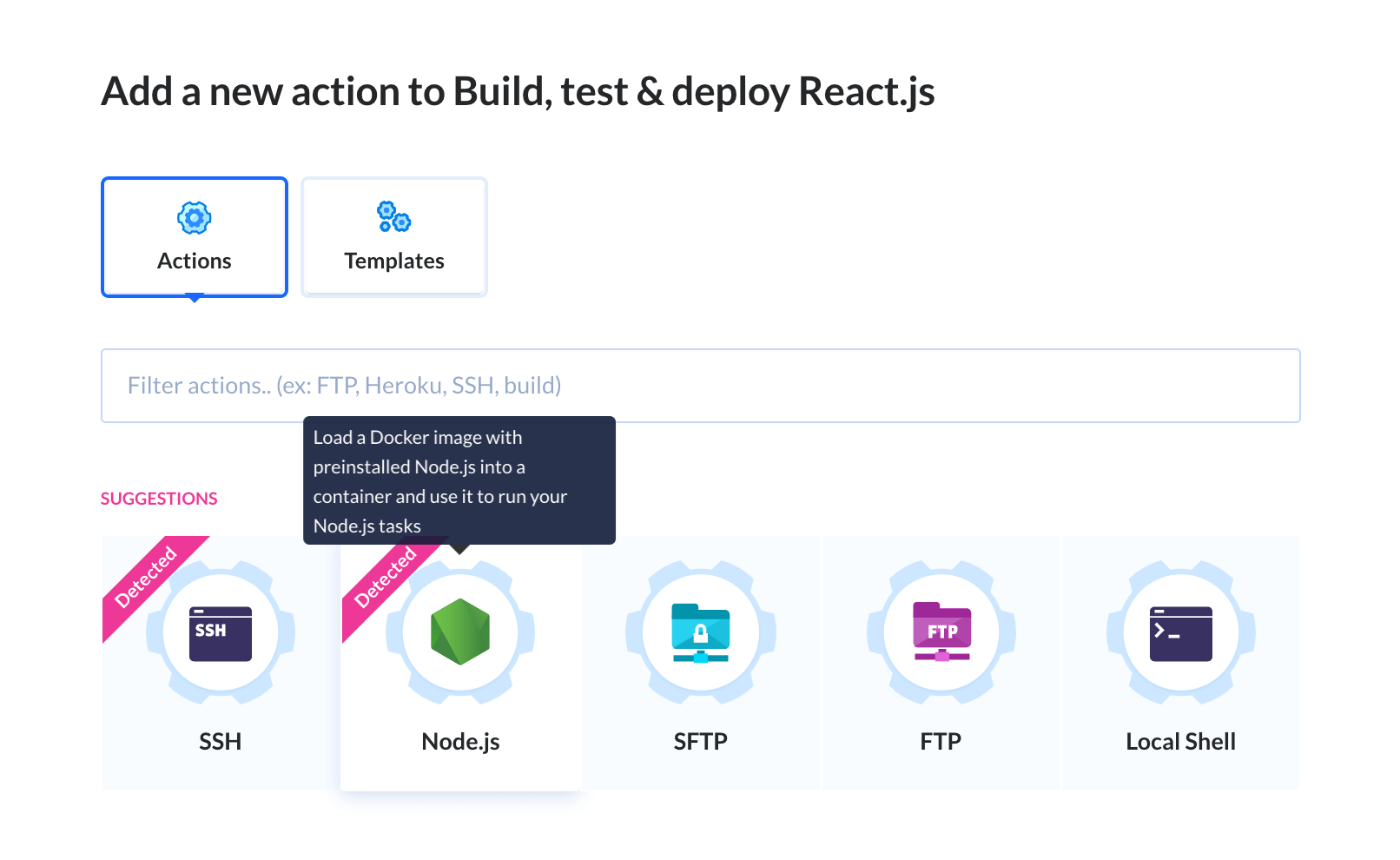This image depicts an interface labeled at the top left with the text "Add a new action to build, test, and deploy React.js." The interface features two prominent buttons situated towards the upper section. The first button, located on the left, is labeled "Actions" and is adorned with a gear icon above the text. This button is outlined in blue, signifying its selection. Adjacent to the "Actions" button is the "Templates" button, which resembles a tab. The "Templates" button has a box shape and clicking it reveals an underlying menu. Above the "Templates" text, there is an icon consisting of three interlocking gears.

Below these two buttons, there is a noticeable space followed by a horizontal bar. Inside this bar, the text reads "Grief, Little Grief, Light Grief, on Filter Actions." Further down, another space is present before the appearance of five circular icons arranged horizontally. Each circle represents different functionalities, labeled respectively as SSH, Node.js, SFTP, FTP, and Local Shell.